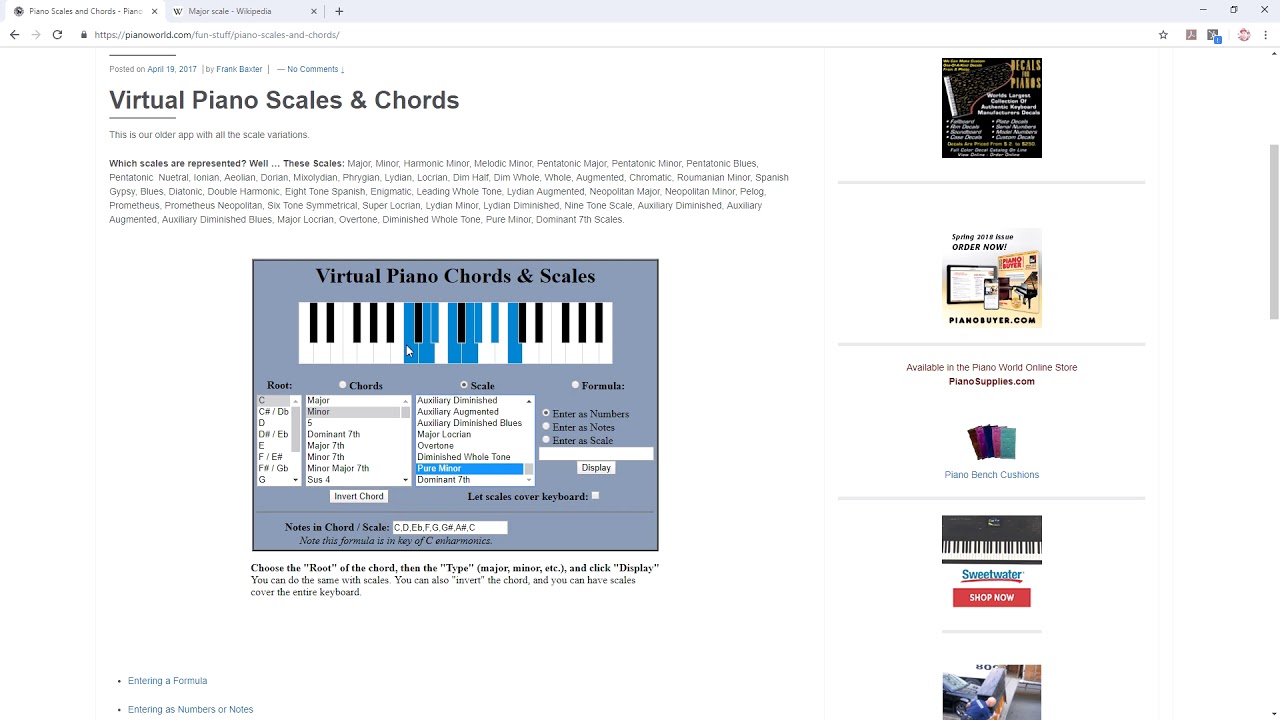Screenshot of a webpage dedicated to piano playing, specifically focused on scales and chords. In the top left corner of the browser, there are two tabs: the first one, titled "Piano Scales and Chords," is selected, and the second one is "Major Scale - Wikipedia." Below the tabs is the address bar displaying the URL "pianoworld.com." Underneath the address bar, there is a post identifier stating, "Posted on April 19, 2017 by Frank Baxter, no comments." The main headline in large text reads "Virtual Piano Scales and Chords."

This page highlights an older version of an app that covers a wide array of scale variations. The scales available include Major, Minor, Harmonic Minor, Melodic Minor, Pentatonic Minor, Pentatonic Major, Pentatonic Blues, Pentatonic Neutral, Ionian, Aeolian, Dorian, Mixolydian, Phrygian, Lydian, and several others.

Beneath the textual information, there is a rectangular image with a gray background. At the top of the image, it reads “Virtual Piano Chords and Scales.” Featured prominently are piano keys, with several highlighted in blue. Below this imagery, the sections for Root, Chords, Scale, and Formula are displayed. For the Root section, "C" is selected. In the Chords section, "Minor" is the chosen chord type. For the Scale section, "Pure Minor" is picked. The Formula section prompts the user to "Enter as Numbers."